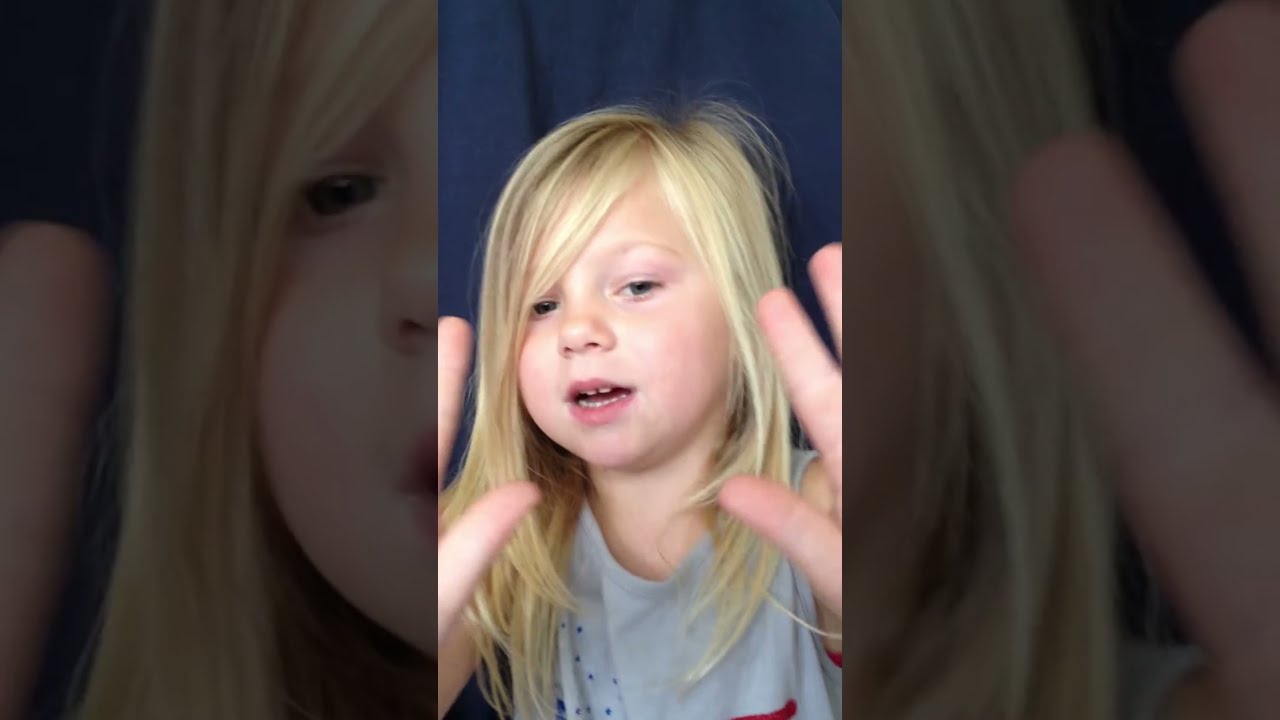This photograph is a composite divided into three vertical sections, with the outer sections displaying darkened, zoomed-in versions of the central image. In the middle, we see a detailed picture of a young girl with fair skin and tousled, straight blonde hair that falls below her shoulders, with long bangs covering one of her green eyes. Her lips are red, and her mouth is slightly open, revealing two teeth, giving the impression that she might be speaking. She wears a grayish tank top with a hint of red and blue accents. The background is a dark navy blue fabric that appears ruffled, adding depth to the image. The girl's face is mostly turned toward the camera, but her eyes glance slightly to her left, contributing to a dynamic, engaging expression.